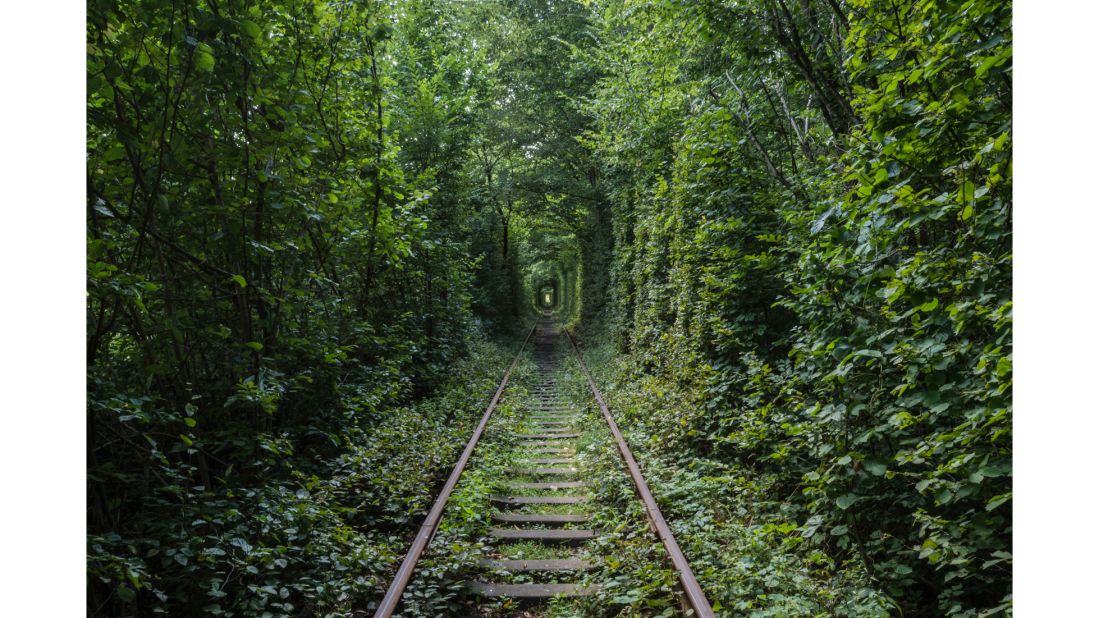A picturesque image captures an overgrown train track cutting through the heart of a lush, green forest. The scene presents a verdant tunnel-like canopy of trees, where the foliage is so dense it forms a continuous archway overhead. The train tracks, primarily wooden ties now partially hidden under a carpet of ivy, grass, and moss, extend away from the viewer, leading into the dense greenery. The track appears to be unused, giving way to nature’s takeover. Small bushes and numerous trees flank the pathway, with overgrowth weaving through the railroad ties. In the distance, a faint, yellowish light peeks through the tree tunnel, suggesting an end to this serene, green passageway. The entire setting is vividly green and brown, exuding a cool, damp atmosphere that feels tranquil and hidden from the bustle of daily life.